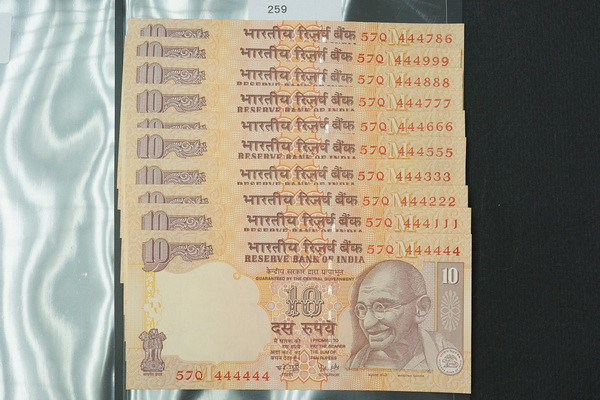The image depicts a slightly yellowish-gold, tan, and light-orange piece of paper that is a denomination of Indian currency, specifically a 10-rupee note issued by the Reserve Bank of India. The note features a black-and-white, side-view image of Mahatma Gandhi, who is wearing glasses, positioned on the bottom right corner. The intricately designed banknote also displays the number '10' adjacent to Gandhi's portrait. Both the upper and lower sections of the note contain serial numbers beginning with '57Q,' followed by combinations of characters like 444444, 444786, and 444999. The text on the bill includes English and another language, presumably Hindi, with "Reserve Bank of India" prominently featured at the top center. The primary note rests upon a stack of similar bills, each bearing unique serial numbers. The background contains a subtle blue on the left-hand side, and the whole scene includes an additional overlay of the number '259' at the top, though it's unclear if this is part of the note or an external addition to the image. The notes appear to be resting on an indeterminate surface, possibly plastic.